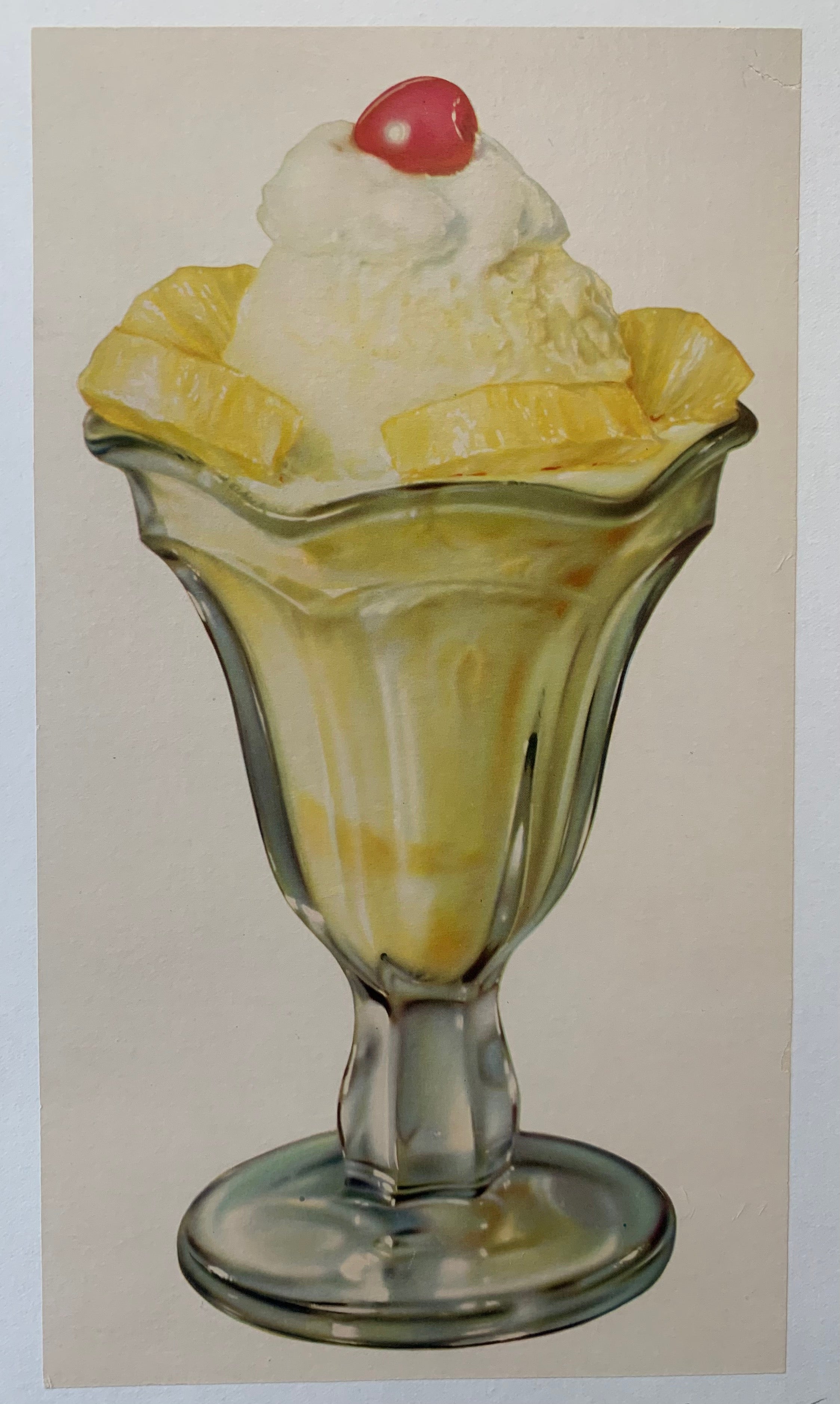The image features a detailed, hand-drawn depiction of an old-fashioned ice cream sundae, reminiscent of a 1950s malt shop treat. The sundae is presented in a classic, fluted, ribbed glass cup, typical of diner milkshake or sundae servings. The glass, clear and elegant, allows us to see the varying shades of beige and yellow of the ice cream and the likely pineapple syrup within. The focal point is a generous scoop of yellow ice cream sitting in the glass, adorned with a slightly deflated crown of whipped cream. Also, carefully placed around the top edge of the glass are two slices of pineapple on each side, framing the central scoop. Topping off this nostalgic dessert is a single, bright red cherry. The composition is set against an off-white, slightly grayish background that gives the piece a timeless, vintage feel, akin to a colored pencil drawing on beige parchment.